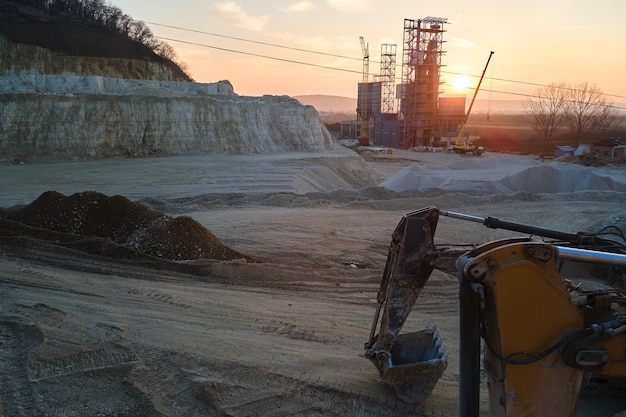This is a realistic and detailed photograph, horizontally oriented, capturing an industrial mining operation during the low light of sunrise or sunset, with the sun near the horizon. The image showcases a strip mine with a vast expanse of sand and dirt, approximately 200 feet wide and long. In the foreground, at the bottom right, there is a partially visible yellow excavator or backhoe with its bucket resting on the ground. The foreground also features dirt and sand spread across the area.

On the left side, a terraced hillside, part of the strip mine, reveals successive layers dug away over time, with some trees adorning the top. In the mid-ground, the mining facility includes towering structures: a yellow crane, metal scaffolding stairs, and additional heavy equipment, predominantly yellow. In front of these structures are more yellow heavy equipment and piles of sand and dirt. There are also power lines running through the site.

To the far right of the image, further in the distance, a pile of white minerals or rocks is visible. The background features gentle hills or mountains and a sky painted with the warm hues of the setting or rising sun. Near the upper right corner of the photograph, spreading trees shade a few small buildings or sheds nestled underneath. The overall scene is an intricate display of a bustling mining operation framed by the natural beauty of the surrounding landscape.